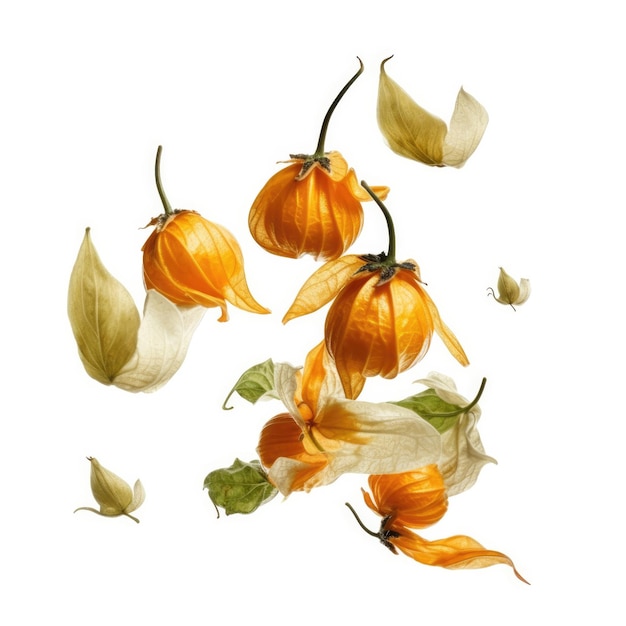The image is a detailed graphic on a white background, depicting various botanical elements evocative of fall. At the center, there are several flowers with closed orange petals, attached to dark green stems, and curiously positioned upside down. Surrounding these flowers are an assortment of leaves in tones of light green, dark green, and yellow. Some yellow leaves appear to have fallen towards the ground, while smaller green leaves seem to be gently drifting. Among the plants, there are also round orange fruits with a peel-like texture, resembling tangerines or small oranges, adding a touch of richness to the autumnal theme. Overall, this artwork, with its muted colors and detailed foliage, seems ideal for fall-themed decorations or a seasonal festival.